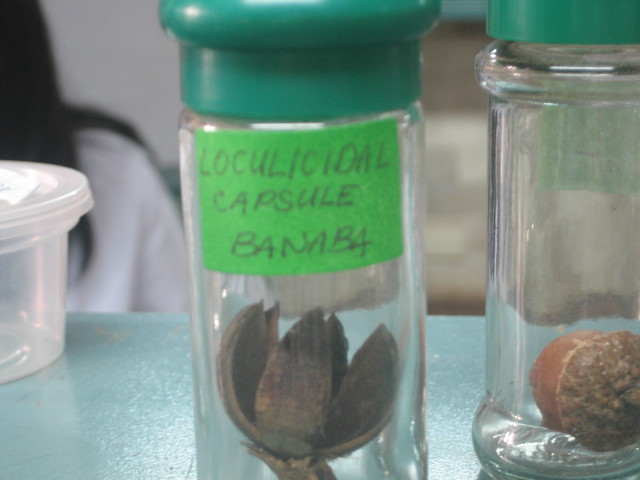This photograph, taken inside a laboratory, showcases two upright glass vials placed on a light bluish-green tabletop. Each vial is sealed with a green lid, though the lid on the vial to the right is shorter. The left vial features a green label with handwritten text in blue ballpoint pen reading "Locally Sedile Capsule Banaba," containing what appears to be a brown, flower-like specimen. The right vial houses an acorn and lacks a label. To the left of these vials is an empty, clear plastic container. In the background, a woman with long, dark hair, clad in a white lab coat, is partially visible, adding context to the scientific setting.